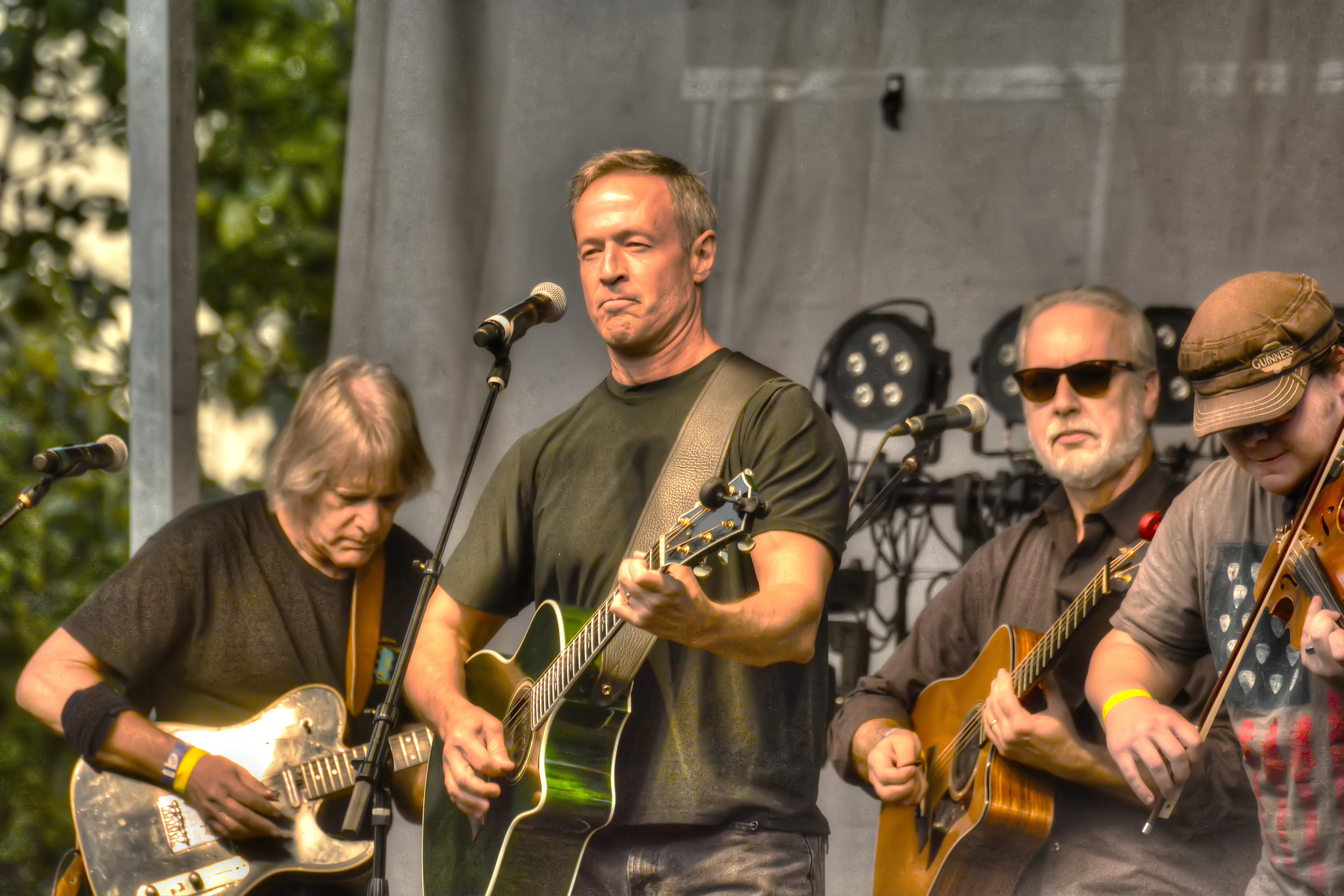The image depicts an outdoor performance featuring a group of musicians on stage, framed by a black canvas backdrop typical of an outdoor festival. Central to the scene is a man who appears to be in his early 40s, wearing an army green t-shirt and jeans. He stands as the lead vocalist, singing into a microphone while playing a green acoustic guitar. To his left, another guitarist with longer gray hair, also dons an army green t-shirt and plays an electric guitar. Behind the lead, on the left side of the stage, another older guitarist, characterized by his short gray hair, dark sunglasses, and gray beard, is seated and playing his acoustic guitar. This guitarist is dressed in a brown button-down long-sleeve shirt. Additionally, on the far right of the stage, a musician with a hat and a brown t-shirt featuring an American flag design performs on the violin.